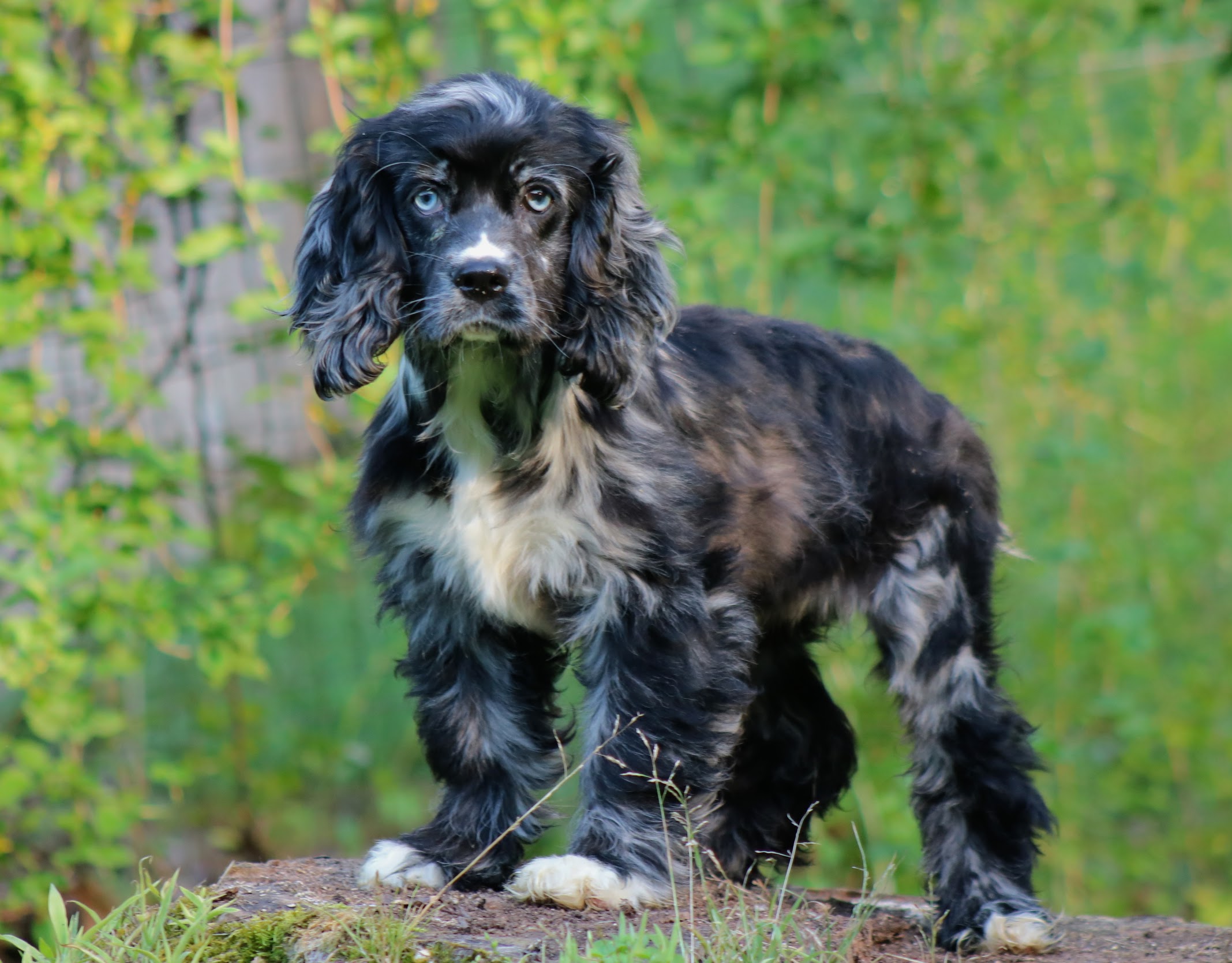This photograph captures a small, possibly older dog, standing proudly atop a large brown rock in an outdoor setting. The dog, likely a mixed breed, has a distinctive speckled coat of black, grey, and white, with particularly shaggy and curly fur that gives it a somewhat unkempt appearance, suggesting it may be in need of a haircut. Its blue eyes, which have a tired look, gaze directly at the camera, creating a captivating focal point. The dog's ears are large and floppy, extending a couple of inches below its chin, and its black nose and white whiskers are clearly visible. Both front paws and its chest feature prominent white fur, with a long white stripe stretching up to the base of its neck. Standing on all four legs, the dog exudes a sense of alertness and curiosity. The background, though blurred and out of focus, reveals a lush, bright outdoor environment with a mix of green grass, thin trees, and tall bushes, indicating that the photograph was taken during daytime. The focus remains solely on the dog, highlighting its unique features and gentle demeanor.